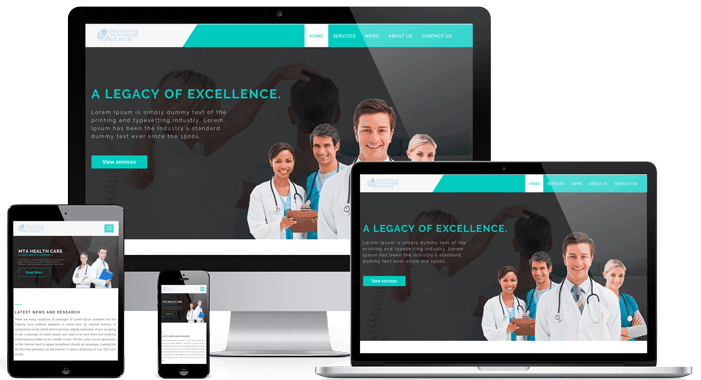The image is a landscape-oriented composition with a stark white background, featuring four electronic devices, each displaying the same webpage. Starting from the lower left corner, there's a tablet positioned in portrait mode. Next to it is a smartphone, also in portrait mode. In the center, behind these two devices, stands a large monitor on a stand. To the right, there's a laptop. 

All the devices showcase an identical website. The highlighted selected tab on the webpage is "Home," with other tabs labeled "Services," "News," "About Us," and "Contact Us." The website displays a gradient banner starting from white in the upper left corner to a shade of seafoam. Below the tabs, the central text reads "A Legacy of Excellence," accompanied by a green button and images of medical professionals.

Intricately, the entire scene underscores the consistency across various devices, emphasizing the website's responsive design in a clean, minimalistic setting.